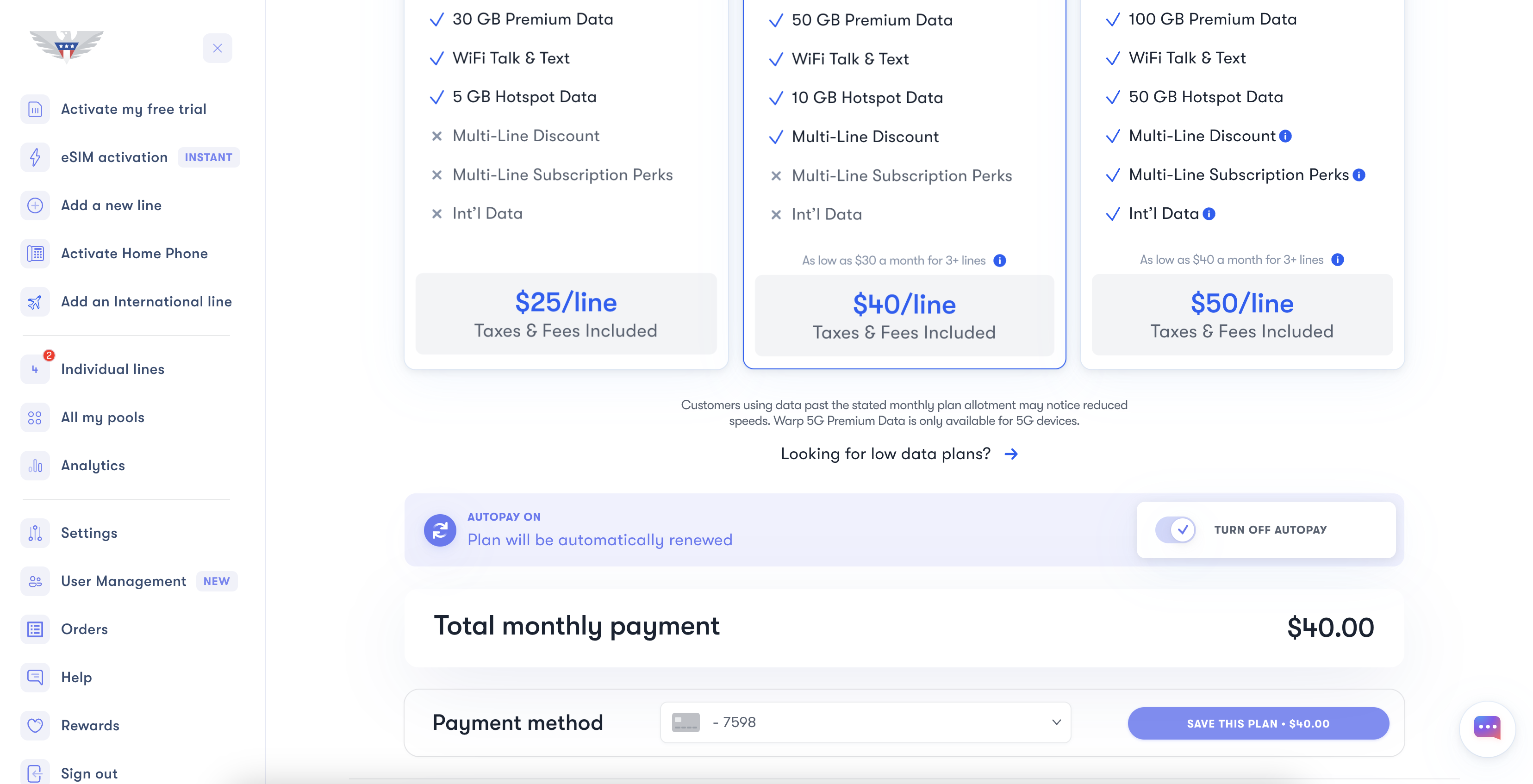The image depicts an interface related to cell phone plans. On the left-hand side, a vertical menu lists various categories including "Activate My Free Trial," "SIM Activation," "Add a New Line," "Activate Home Phone," "Add an International Line," "Individual Lines," "All My Pools," and "Analytics." Additional options at the bottom of this menu include "Settings," "User Management," "Orders," "Help," "Rewards," and "Sign Out."

In the main section, three cell phone plans are displayed. The first plan costs $25 per line and is highlighted in blue. The middle plan costs $40 per line, also in blue. The third plan is priced at $50 per line, again highlighted in blue. Each plan includes a list of benefits marked by check marks and X's to indicate which features are included and which are not.

Beneath the plans, a prompt asks, "Looking for low data plans?" accompanied by a blue arrow pointing to the right. Below this, there's a note stating that "Auto pay on plan will be automatically renewed," with an option to the right to "Turn off auto pay."

Further down, the interface shows the "Monthly total monthly payment" in black, indicating a selected payment of $40. There is an option to "Save this plan." In the bottom right corner, a blue and purple chat icon is visible for customer support.